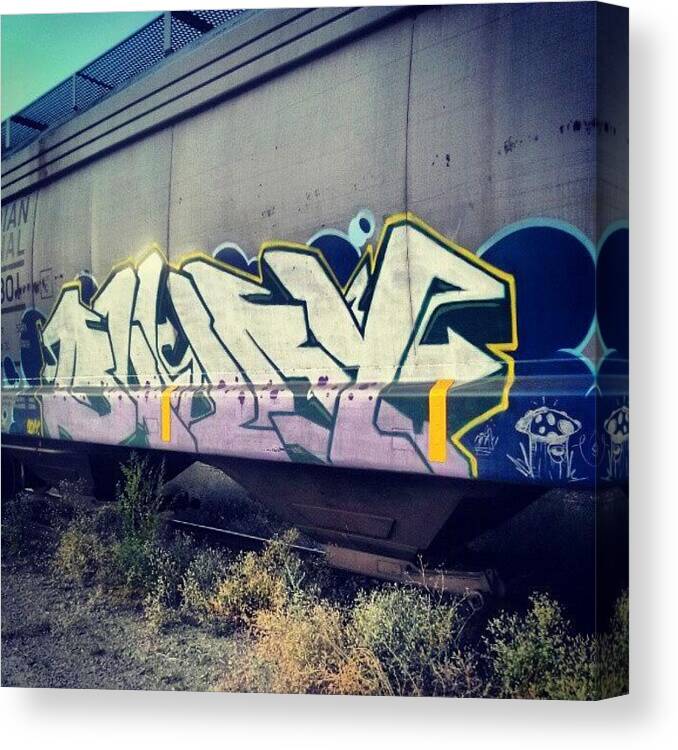The image depicts a stationary, steel-gray rail car adorned with intricate graffiti. The train car sits diagonally in the frame, extending from the center right to the center left. The graffiti showcases entangled white bubble letters with lilac-colored lower halves, outlined in yellow, and accompanied by a dark drop shadow effect. A dark blue section of the train features what appears to be a chalk-like drawing of a mushroom on the far right. Below the train, overgrown weeds, browned from neglect and sporadically interspersed with patches of green, rise almost to the base of the car, indicating that it hasn't moved in quite some time. Visible beneath the train is a piece of track, partially buried under the encroaching foliage. The scene resonates with a sense of abandonment, highlighted by the dry, overgrown environment around the rail car.